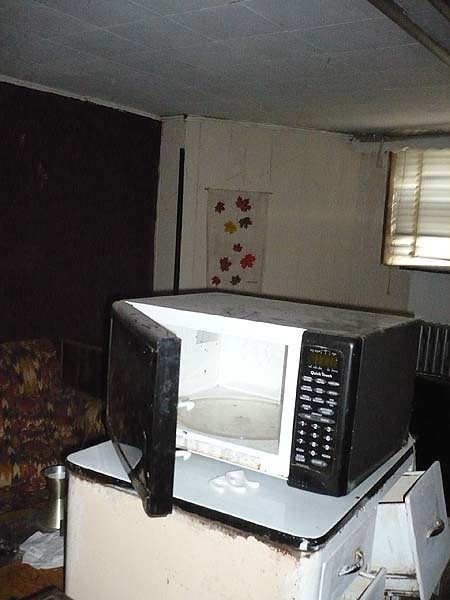In this rundown room, likely part of an old apartment or rec room, the image captures the state of neglect and decay. Dirty white walls and ceilings frame the space, while a small, beat-up window is dressed with tattered blinds. To the left of this window, a curved wall features a multi-colored leaf decoration. Below the window stands a broken white desk or kitchen cart with several drawers awkwardly open, revealing its age. Atop the cart sits a dusty black microwave, its door wide open. Adding a splash of color to the otherwise drab room is an old couch with a vibrant, retro pattern in shades of red and yellow, reminiscent of designs from the 60s or 70s. The overall scene depicts a room that has seen significantly better days.